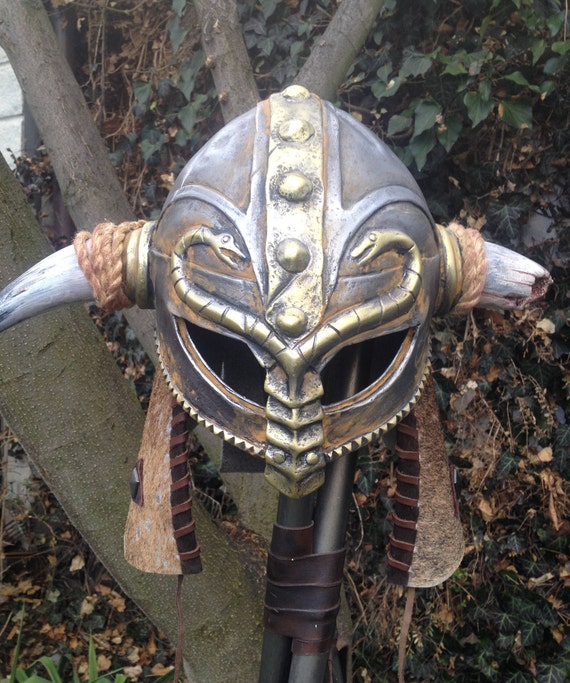This photograph depicts an ancient bronze war helmet mounted on a staff or spear. The helmet features intricate detailing with two intertwined snakes above the eye slits, each snake's head facing the other, forming an almost heart-like shape. The snakes, cast in gold, add a dramatic contrast to the overall silver tone of the helmet. Running along the centerline from the bridge of the nose to the back of the head are five large brass rivets.

On either side of the helmet are horns made from natural animal horn with a rope tied around them. The right horn is notably broken off about halfway, showing additional cracking towards the helmet's base, while the left horn remains intact but partially obscured. The eye slits are shaped similar to cat eyes, and the nose piece has layered designs leading up to the point where it transitions into the snake motif. There are decorative round spots along the helmet, adding to its ornamental appeal. The bottom edge of the helmet, circling around the cheeks, is serrated in a zigzag pattern.

On the back sides of the helmet, a piece of striped leather cloth dangles down, possibly meant to protect the neck. The background of the picture features a close-up view of a hillside covered in English ivy, with the quadruple trunk of a small tree presenting a natural, rustic setting. The makeshift stand, formed by two staffs taped together with electrical tape, completes the display of this detailed and well-preserved historical artifact.